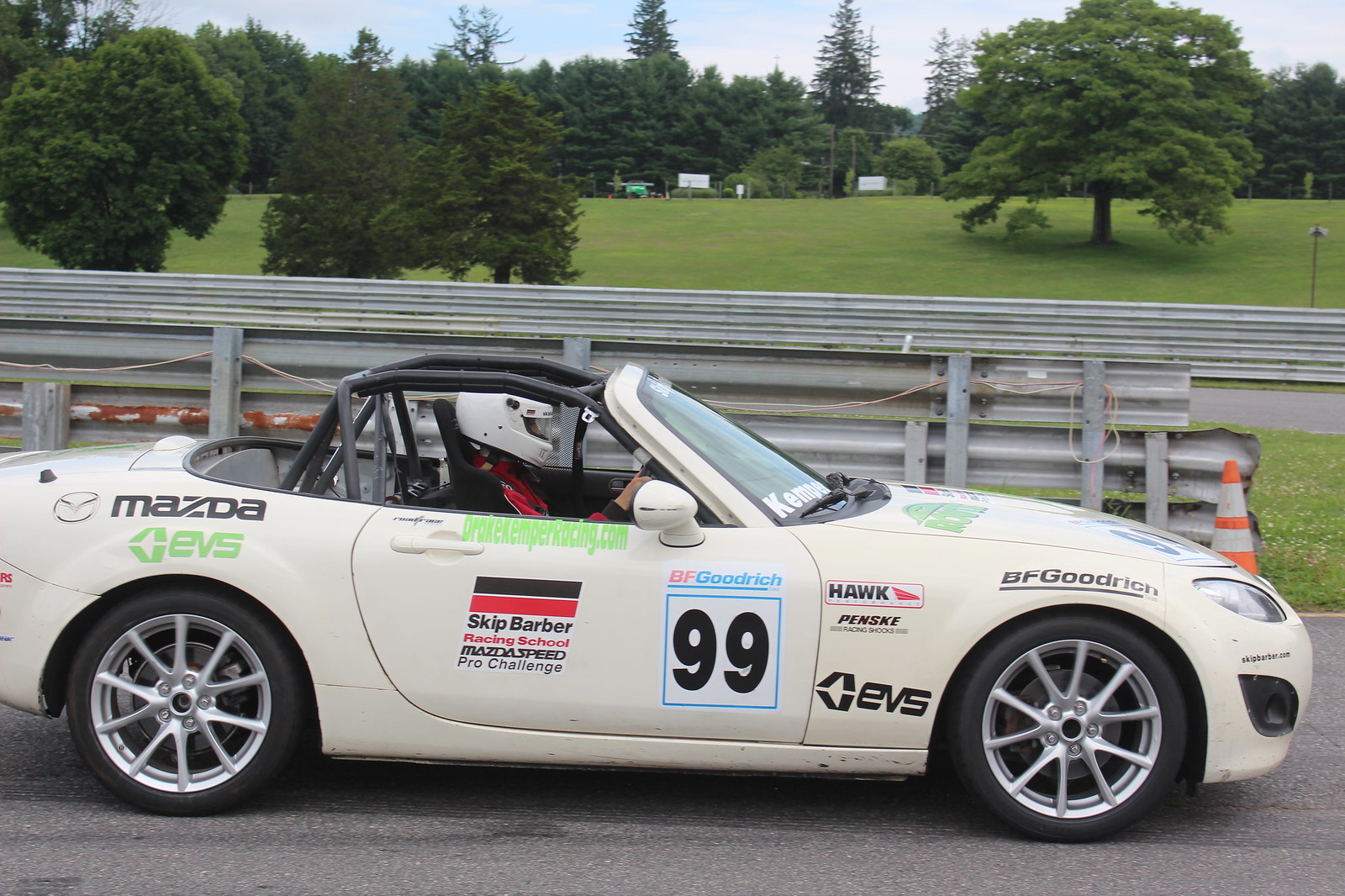The image depicts an old-school Mazda EVS race car, stationary on a racetrack, though it appears frozen in motion due to a high shutter speed. Positioned sideways in the frame, the car prominently displays various logos, including those of Skip Barber Racing School, BFGoodrich99, Hawk, Penske, and Mazda Speed Pro Challenge. The background features multiple metal guardrails typical of racetracks, a patch of grass, and an orange and white traffic cone adjacent to the car. In the further distance, there are a few short trees under a cloudy sky, with little to no sunlight visible.